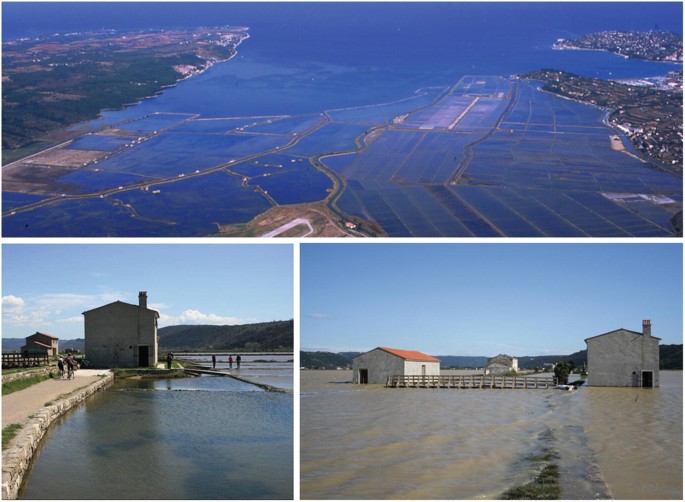This is a composite panel featuring three distinct photographs that capture various scenes of nature and human structures. The top photograph provides an aerial view of a waterway, likely a lagoon, which is flanked by multiple islands on either side and converges into a larger body of water, such as an ocean or sea. The water is notably blue, and the wetlands extend almost to the lagoon's mouth. In the top left corner, a small concrete building with a chimney and a little fence in front appears to be surrounded by water, suggesting potential flooding.

The bottom two photographs offer ground-level views. The first of these shows a barn or house situated by a small body of water, possibly a river, lake, or creek. The scene features a clear blue sky with a couple of clouds, a bridge in the background, a hillside, and a walkway, presenting a serene environment. The second ground-level image highlights brownish water surrounding a plain, concrete building similar in style to the one in the aerial shot; a fence is visible in the background. This image suggests flooding, as the walkway depicted in the "before" photo, once dry and populated by people, now appears submerged. All three photographs are taken during daylight under blue skies, drawing a vivid picture of natural landscapes intersected by human-made structures, some of which are seemingly battling the encroaching waters.